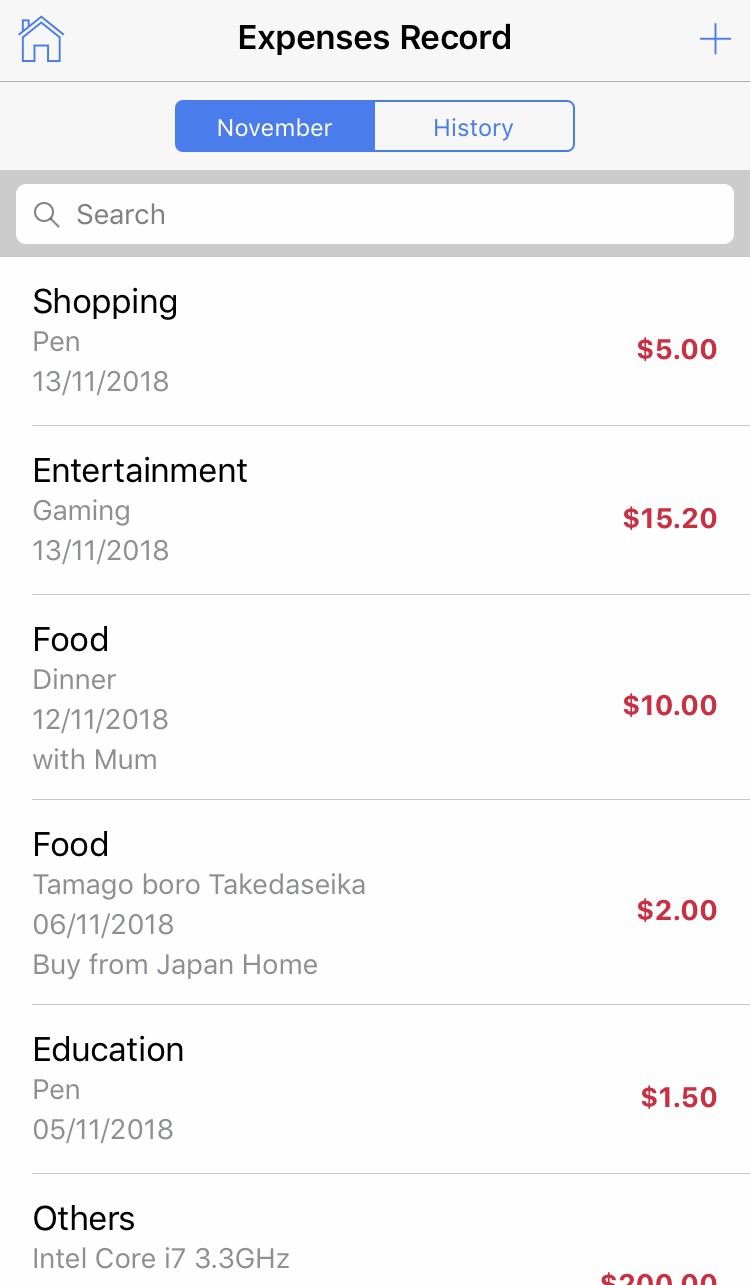The image appears to show a smartphone screen in portrait mode, likely an iPhone due to its interface design. At the top of the screen, there is a black bar with the text "Expenses Record." On the left side of this bar is a small blue icon depicting a house, and on the right is a blue plus symbol. 

Directly below this bar are two buttons. The first button on the left is blue with the text "November" in white, while the button on the right is white with the text "History" in blue. Beneath these buttons, there is a white search field with a magnifying glass icon and the placeholder text "Search," all enclosed in a gray box.

The main section of the screen consists of multiple fields organized in a list, each separated by thin gray lines. The first field shows an entry labeled "Shopping" with a date of "13/11/2018" and an expense amount of "$5" in red. The next field is labeled "Entertainment," specifying "Gaming" with the same date and an expense of "15.20."

Following this, there is a "Food" category, listing "Dinner with mom" and an expense of "$10." Another "Food" entry lists "Tamago Borotakedaseika," described as "buy from Japan home" with an expense of "$2." 

Next is an "Education" category entry for a "pen" priced at "$1.50." Lastly, there is an entry under "Others" for an "Intel Core i7 3.3GHz" processor, though the expense amount is cut off and not fully visible.